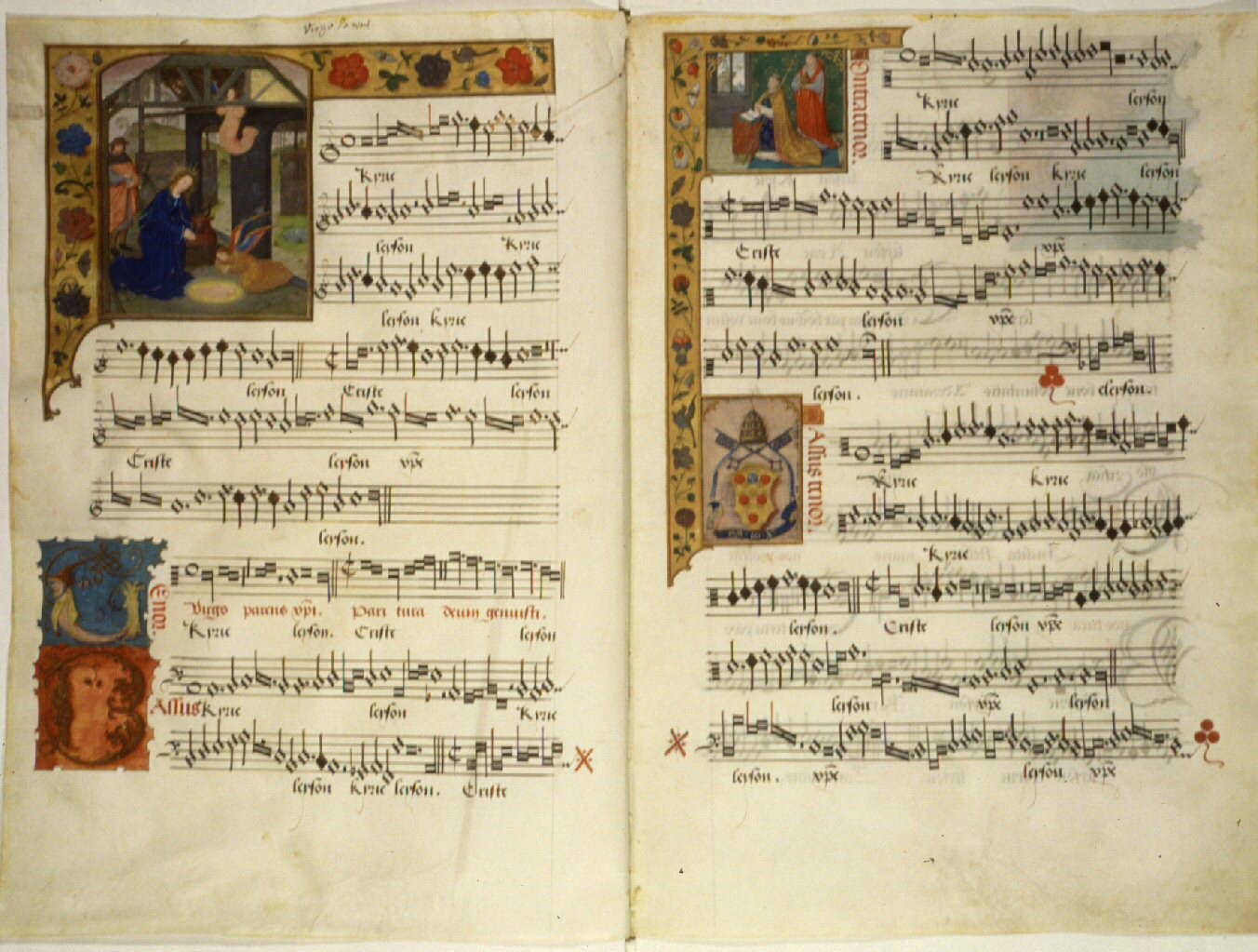This image is a detailed photograph of two pages from a medieval musical manuscript, probably dating back to the Middle Ages. The top left-hand corner of the first page features a beautifully illustrated scene of the Annunciation, depicting an angel kneeling in front of the Virgin Mary. The Virgin Mary is adorned in a black robe and is in a bending position, while the angel stands out in a brown robe with striking, rainbow-colored wings. The musical text, written in Gothic print, includes various notations with recurring letters such as K-R-U-Z-E, F-A-F-O-N, K-Y-Z-I-E, and L-A-F-O-N-K-Y-Z-I-E mingled throughout the musical staffs that span the page.

On the opposing page, another intricate illustration graces the top left-hand corner, showing a person in a red robe standing behind another individual cloaked in black with a gold cape, both looking outward. Similar Gothic lettering, including sequences like K-Y-Z-I-E and F-O-R-F-O-Y, intertwines with the musical notes. The manuscript's notes also feature words below them, indicating a vocal component to the music. The pages display signs of aging, with the paper having a beige-tan tone and some oxidation. The vibrant color palette of the illustrations includes reddish oranges, blues, greens, blacks, grays, and whites, adding to the rich and historical essence of this religious music manuscript.